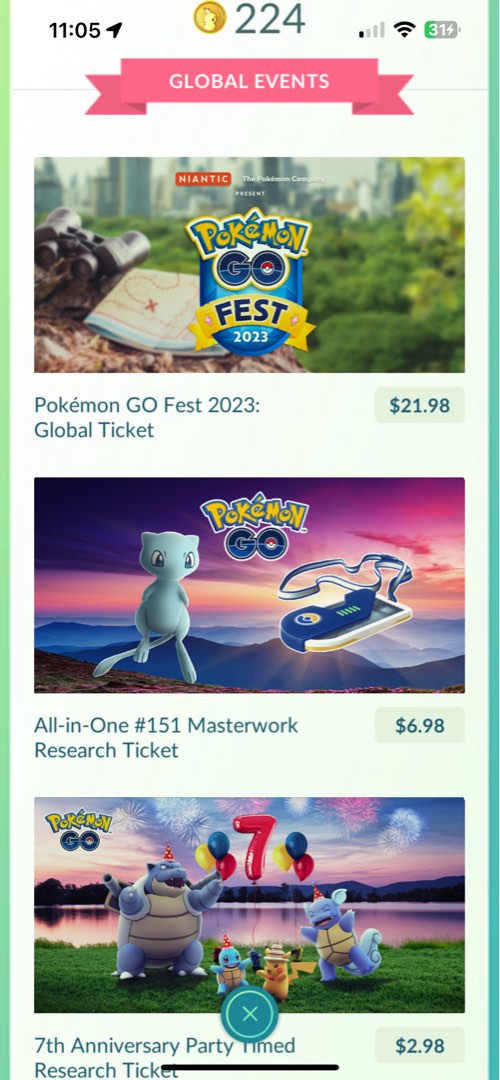The image is a screenshot from the Pokémon GO app, captured at 11:05 while the phone was charging and had 31% battery remaining. Prominently displayed at the top center is a small gold coin symbol accompanied by the number 224. Below this, a ribbon banner with pink and white text reads “Global Events.”

The main section of the image features three distinct tiers, each advertising an event ticket:
1. The top section promotes the “Pokémon GO Fest 2023 Global Ticket” priced at $21.98, with relevant Pokémon illustrations.
2. The middle section highlights the “All-in-One #151 Masterwork Research Ticket” for $6.98, also adorned with themed Pokémon artwork.
3. The bottom section advertises the “7th Anniversary Party Timed Research Ticket” for $2.98, featuring another set of Pokémon graphics.

Near the bottom center of the image, a blue circle with a white 'X' is visible, likely indicating a button to close or dismiss a popup or menu.